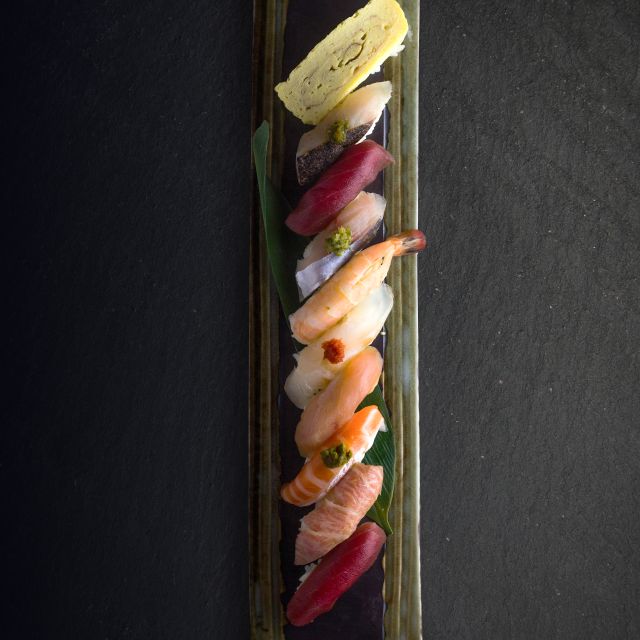The image showcases an assorted sushi platter against a charcoal-black background. The sushi is meticulously arranged on a long platter with golden ends, atop a dark brownish-green surface resembling bamboo, and a green leaf extending underneath the sushi pieces. The platter features a variety of nigiri, each distinctly different in color and texture. 

From top to bottom, the selection includes tamago, a sponge-like yellow egg; a pink fish with a triangular piece of darker skin and a dab of wasabi; deep red magura (tuna); mackerel with a soft pink interior and silver exterior garnished with either onions or wasabi; a shrimp with a pink tail; white fish topped with orange; light beige fish with red at the tip; salmon with orange and white stripes and a touch of wasabi; and fatty tuna with prominent white fat marbling into a light pink hue. The detailed assortment and vibrant colors reflect an artistic and carefully crafted presentation of raw seafood.